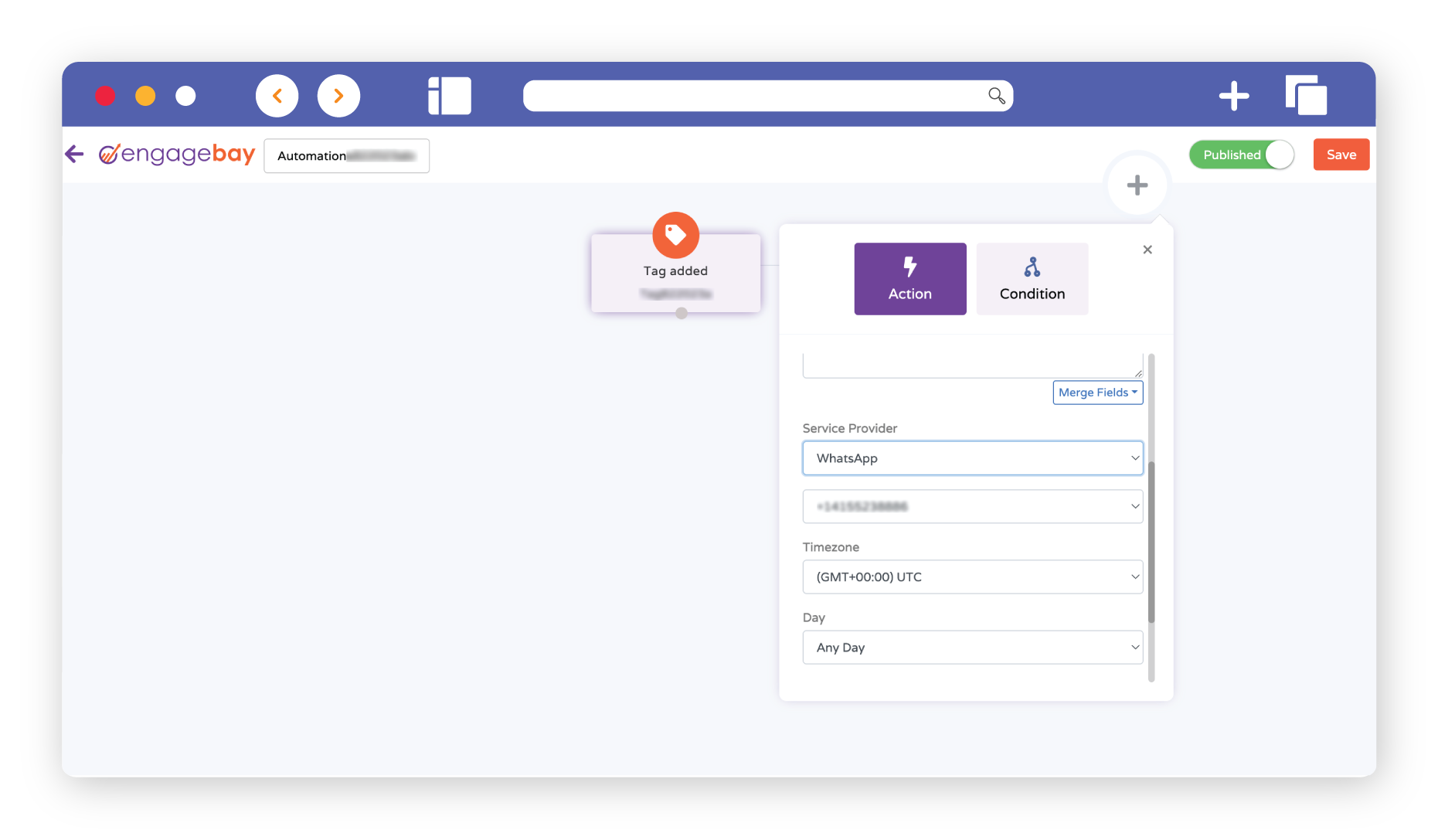This image is a snapshot of an Engage Bay interface tailored for our website page. At the top of the interface, navigation icons for forward, back left, and right are prominently displayed, along with a search bar featuring an hourglass icon, a plus sign, and an additional, unidentified icon. Below this top navigation, the Engage Bay logo is paired with a distinctive purple arrow, reinforcing the brand's visual identity.

To the left side, there is a box labeled "automation," partially redacted to obscure additional text. On the far right side, a green button marked "Published" in white font stands out, indicating the current status of a document or item. Next to this, another button appears in red, also with "Save" printed in white, providing a clear actionable option.

Centrally located on the page, there's a red-tagged box with a "tag added" label clearly visible, ensuring users can easily track tagging actions. Adjacent to this, another box includes a purple "action" label and a white "condition" label, with "merge fields" mentioned below, defining further conditions and actions within the automation process. 

Towards the bottom, another segment has a label for "Service Provider," listing WhatsApp as the selected service. Below this, a partially redacted box is followed by time zone details: "GMT," "no time," and "UTC." Lastly, another box specifies "Day," with "any day" chosen as the input, completing the detailed layout of this Engage Bay interface.